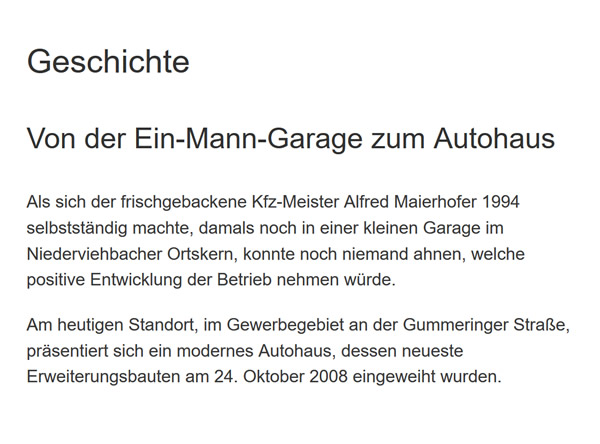This horizontal image is a black-and-white poster or sign with no border, featuring German text. Dominating the upper left corner in larger letters is the word "Geschichte," followed by "Wander-Ein-Mann-Garage-Zum-Otto-Haus" in the same size. Below these prominent titles, there are two paragraphs of smaller text. The first paragraph includes a visible date, 1994, possibly providing historical context or explaining something about a garage or car sales place. The second paragraph consists of only three lines. The entire image has a minimalistic design with the black text printed on a white background, placed centrally and occupying most of the visual space, emphasizing the nature of the image as a textual sign or poster.